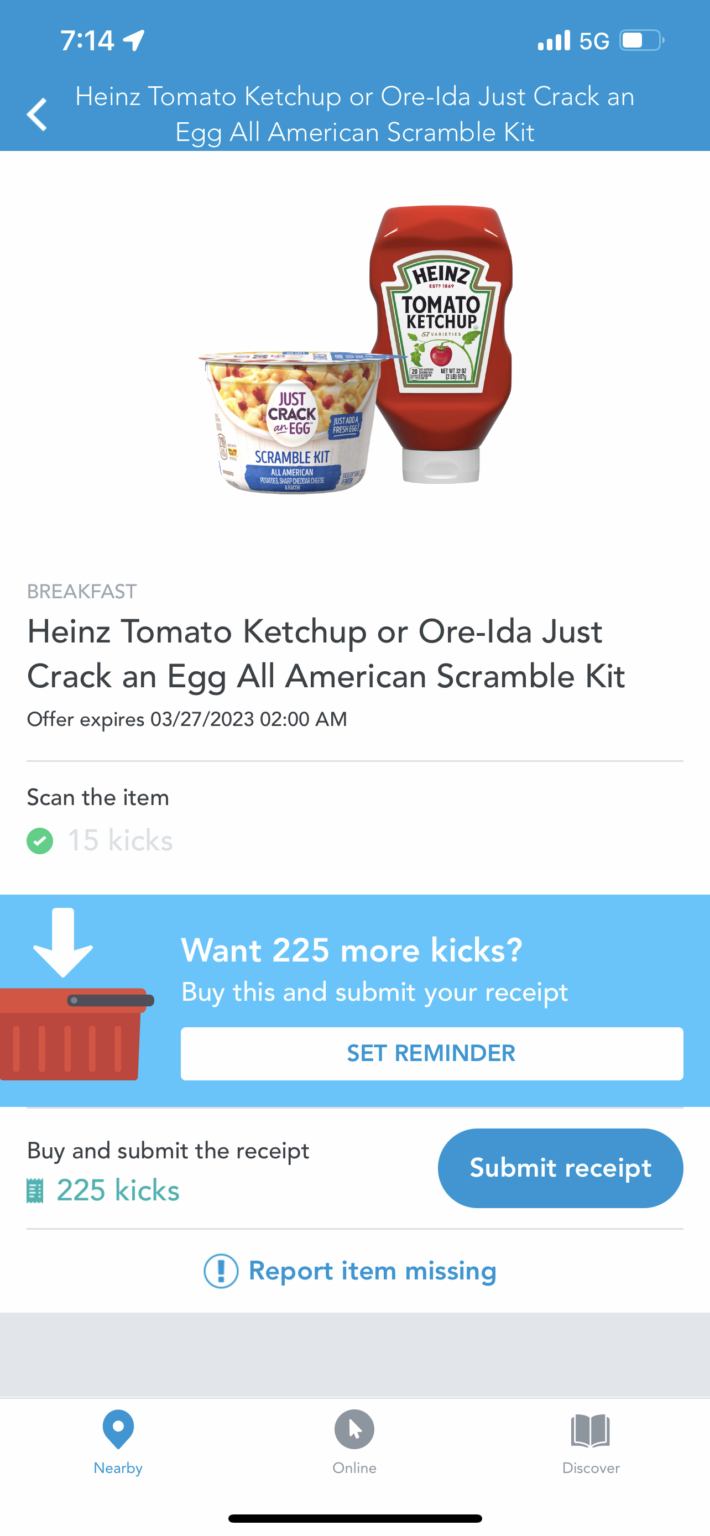The image shows a screenshot of a product listing on a user's phone, displaying two grocery items: Heinz Tomato Ketchup and Oura Ida’s Just Crack an Egg All-American Scramble Kit. At the top of the screen, a wide, bright blue banner displays essential phone information: the time is 7:14, there is a 5G network with full bars, and the battery is at about 60%. Below this banner, in white text, the names of the products are prominently displayed: "Heinz Tomato Ketchup or Oura Ida Just Crack an Egg All-American Scramble Kit."

The main content area features images of the products: a full bottle of Heinz Tomato Ketchup and a cup labeled "Just Crack an Egg Scramble Kit." Underneath the images, in light gray capital letters, the word "BREAKFAST" is displayed, followed again by the product names in black text.

Further below, in gray text, instructions are given: "Scan the item," accompanied by a green circle with a white checkmark. To the right, in light gray text, it indicates that scanning the item will earn "15 kicks." 

A sky-blue horizontal box follows, containing the text "Want 225 more kicks? Buy this and submit your receipt," in white. Inside this box is a white button with the text "Set Reminder" in bright blue. Below this, on a white background, further instructions to "Buy and submit the receipt" are provided, with "225 kicks" highlighted in bright blue. To the right of this, a darker blue button says "Submit Receipt" in white text.

At the bottom of the screen, a bright blue icon of an exclamation point within a circle directs users to "Report item missing," also in bright blue text.